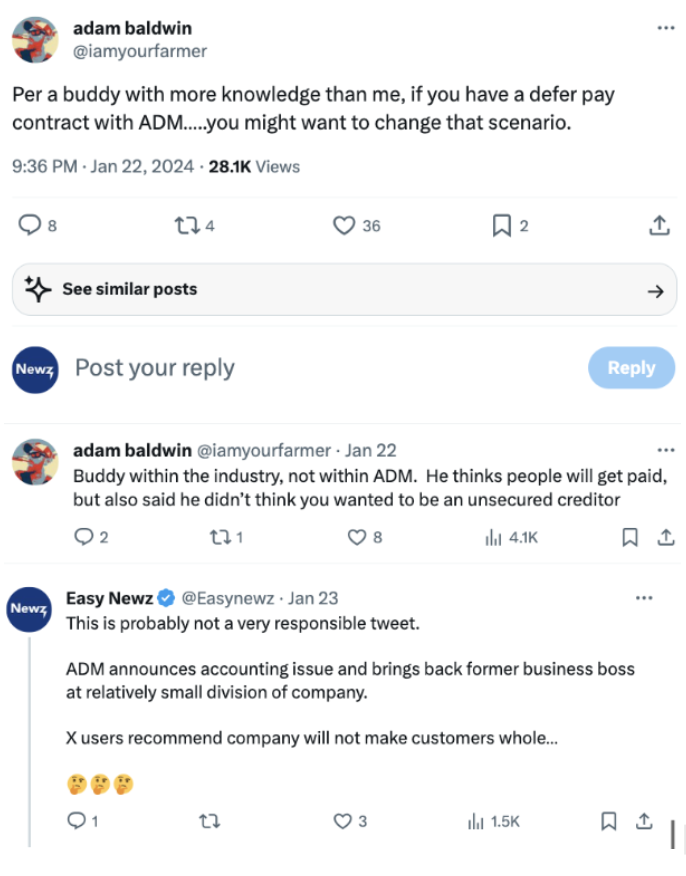This caption is referencing a Twitter post by the user Adam Baldwin, who tweets under the handle "I am your farmer." The post, made on January 22, 2024, at 9:36 PM, addresses concerns regarding deferred pay contracts with ADM (Archer Daniels Midland Company). Baldwin suggests that individuals should reconsider these contracts based on advice from a knowledgeable source within the industry (but not within ADM itself). The tweet has garnered significant engagement, including 28,100 views, 8 comments, 4 retweets, 36 likes, and 2 bookmarks. In the discussion, Baldwin notes that while payments are expected, he expresses reluctance to become an unsecured creditor. The news outlet EZ News commented, criticizing the tweet as possibly irresponsible. They mention that ADM had announced an accounting issue but reassured that, according to former users, the company is unlikely to cause financial harm to its customers.